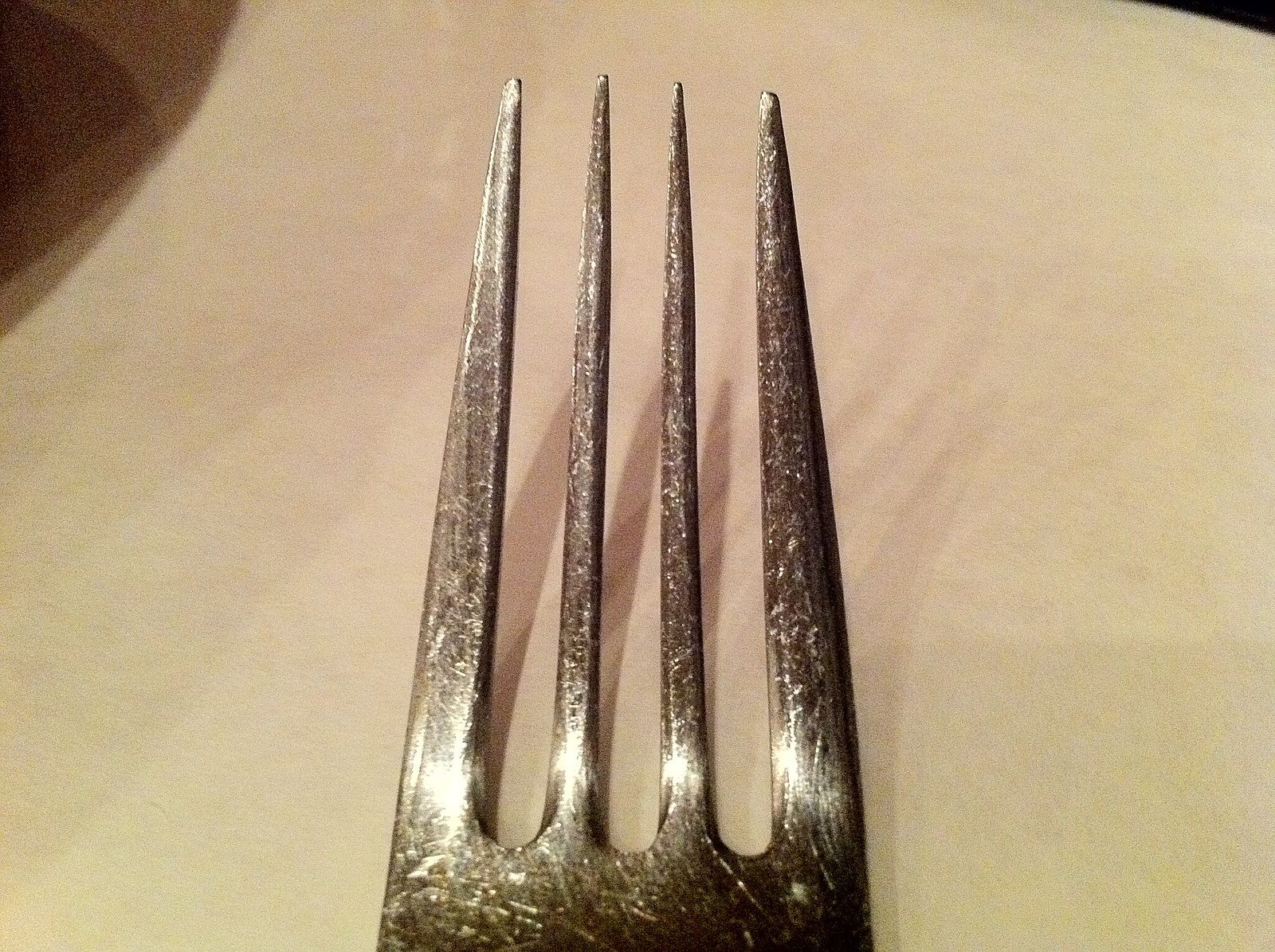The image depicts an up-close view of a well-used silver fork focusing on its four prongs resting on a creamy white, tablecloth-like background with noticeable shadows cast over it. The two end prongs are flatter, while the middle two taper to sharper points. Despite its evident use, indicated by numerous scratches and dings, the fork shines under a light source that casts its reflection and shadows prominently. In the upper left corner, there's a touch of a darker shadow adding contrast to the predominantly bright background. The nuanced lighting enhances the fork's intricate details and lends a slightly brownish-gray hue to its silver surface.